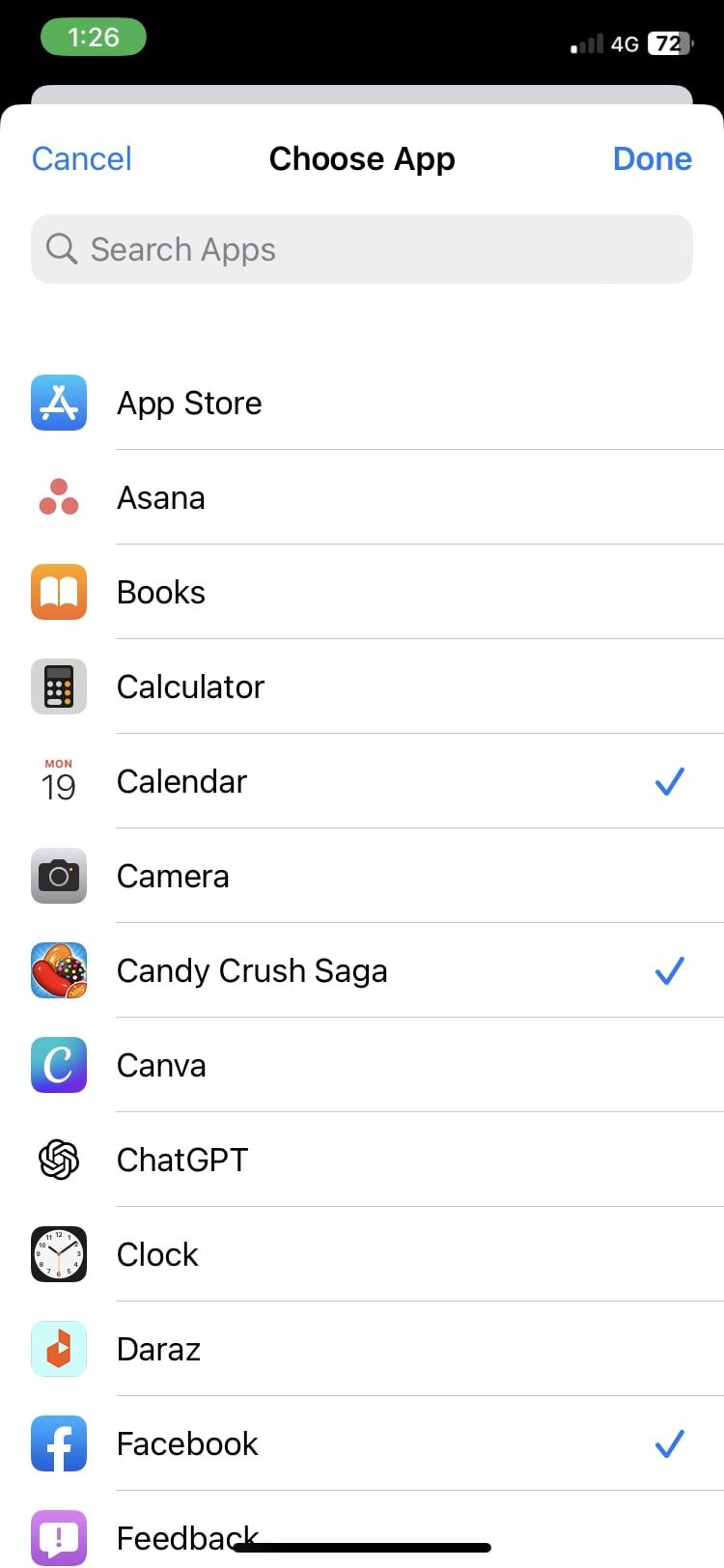The image captures the top section of an iPhone screen. At the very top, the screen features a black background, displaying the time "1:26" in a white font encapsulated in a green bubble towards the left. To the right, the signal strength is low, indicated by a single bar next to the "4G" symbol in white. The battery icon is also visible, showing a 72% charge.

Moving to the main part of the screen, the top-left corner features the word "Cancel" in light blue font with an initial capital letter. Towards the center, the bold black text with initial caps reads "Choose App." On the top-right side, the word "Done" is prominently displayed in bold blue font, also with an initial capital.

Beneath this, there is a grey search bar adorned with a grey magnifying glass icon on the left. Inside the search bar, in light grey text, the words "Search Apps" appear.

Below the search bar, a list of apps is displayed in a vertical arrangement. The apps shown include: "App Store," "Asana," "Books," "Calculator," "Calendar," "Camera," "Candy Crush," and more, each listed in a standard black font.